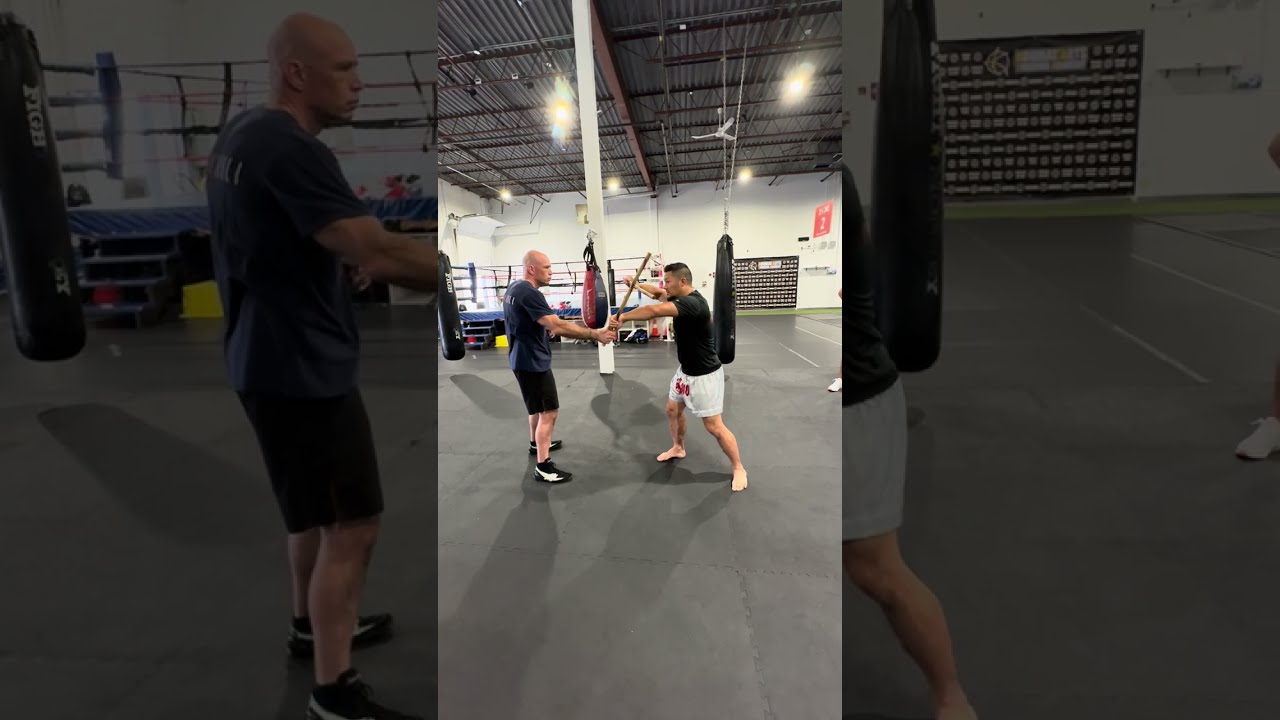The image depicts a scene inside a boxing gym, showcasing two men engaged in what appears to be a stick sparring session. The photograph is centered on the two men, taken from a slight distance. The man on the left wears a navy blue short sleeve shirt, black shorts, and black and white sports shoes. He is bald, muscular, and taller than his sparring partner. The man on the right dons a black t-shirt and white shorts and is barefoot. Both men are gripping long sticks, which they hold up in the air as if in the midst of a training maneuver.

In the background, a boxing ring is visible to the upper left, as well as a punching bag behind the man on the right. The gym itself has a spacious, gray floor, an exposed metal roof with beams and lights, and a white back wall. Notably, the image features a thick border on both sides, created from enlarged and greyed-out elements of the same picture, superimposed to frame the central photograph.